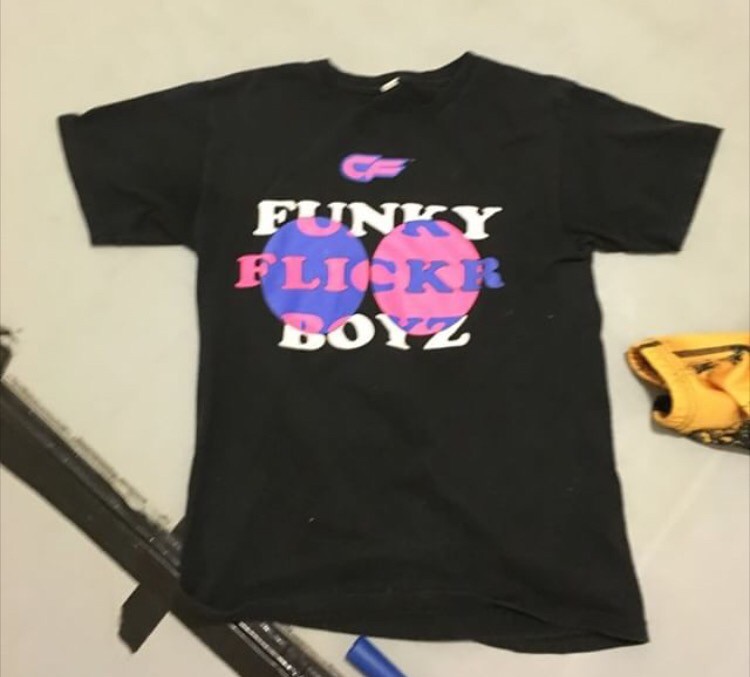Photograph of a black t-shirt meticulously laid out with its arms extended on a pristine white surface. On the right side of the image, a gold-yellow piece of clothing peeks into the frame, adding a touch of contrast. The bottom-left corner features a large, rectangular metal object. The t-shirt's design includes vibrant pink and blue letters "CF" centrally positioned just below the collar. Two circles flank these letters, a blue one on the left and a pink one on the right. The graphic text "Funky Flickr Boyz" arches across the chest area, with the word "Funky" written in white, "Flickr" in blue over the pink circle, and "Boyz" in pink over the blue circle, creating a vivid and dynamic visual effect.